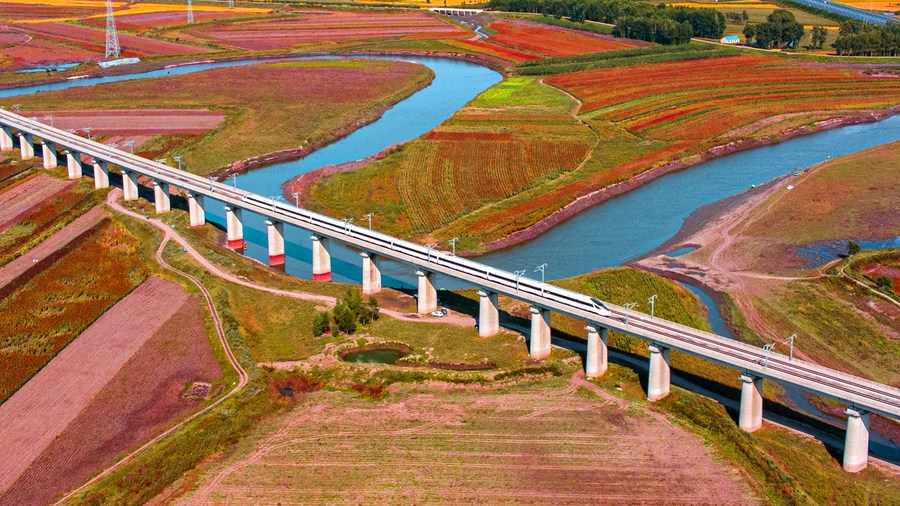The image presents a striking aerial perspective of a modern monorail bridge, running diagonally from the top left to the bottom right. The bridge, supported by numerous white concrete columns, traverses a narrow, winding river that twists from the left, curving around and towards the viewer before veering off to the right. A sleek and advanced white monorail train with a sloped lead car is seen traveling on the bridge, enhancing the futuristic feel of the scene. Below the bridge, the landscape is a patchwork of fields, featuring different colors and patterns, including rows of red, orange, and green hues, indicative of diverse vegetation or farmland. The earth around the waterway is brown, with patches of reddish-brown soil and hints of green grass and sparse shrubs. The top right corner of the image is dotted with trees, adding to the natural scenery. The image’s combination of intricate land and water details with advanced transport infrastructure suggests a blend of nature and human innovation, possibly captured through a meticulously detailed painting rather than a photograph.